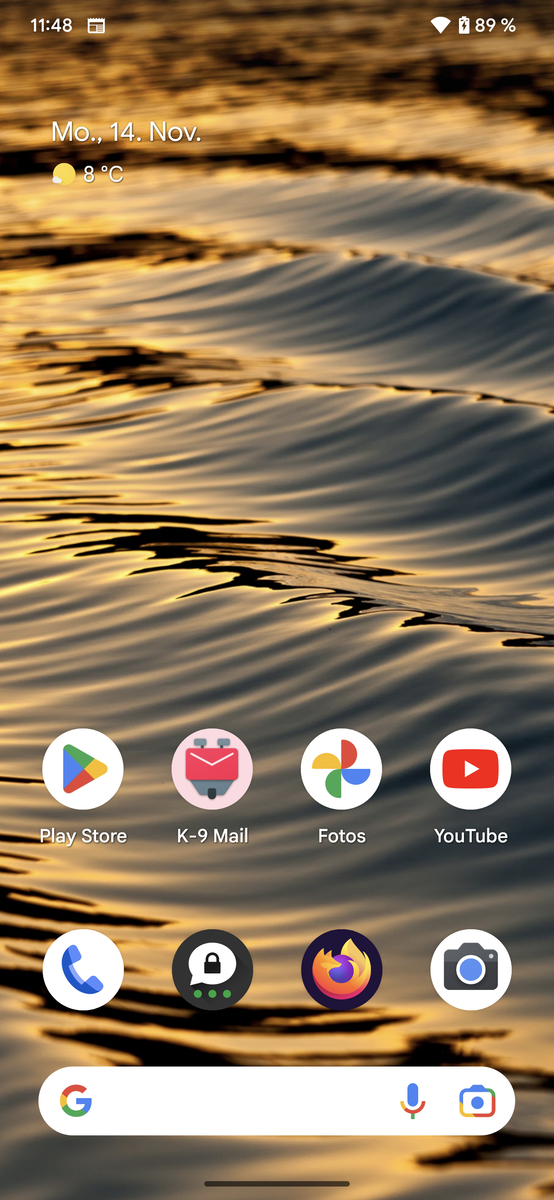The screenshot captured on a smartphone displays the current time of 11:48. At the top, various system indicators are visible, including a Wi-Fi icon and a battery level showing 89% charge. The date is formatted as "Mo... 14.. Nov...," and the weather condition is depicted by a sun partially covered by a small cloud, indicating 8 degrees Celsius.

The central portion of the screenshot features an image resembling waves on the ocean. However, the unique texture created by numerous fine lines gives it an illusion akin to sand dunes. The color palette transitions from a grayish hue on the right side to a golden orange shade on the left and top areas.

Beneath this image, four icons are arranged in two rows. The top row contains icons labeled with their respective app names: Play Store, K9 Mail, Photos, and YouTube. The bottom row shows three more icons without labels, featuring a white circle with a blue phone handset, the Firefox logo, and a white circle containing a camera icon in the middle.